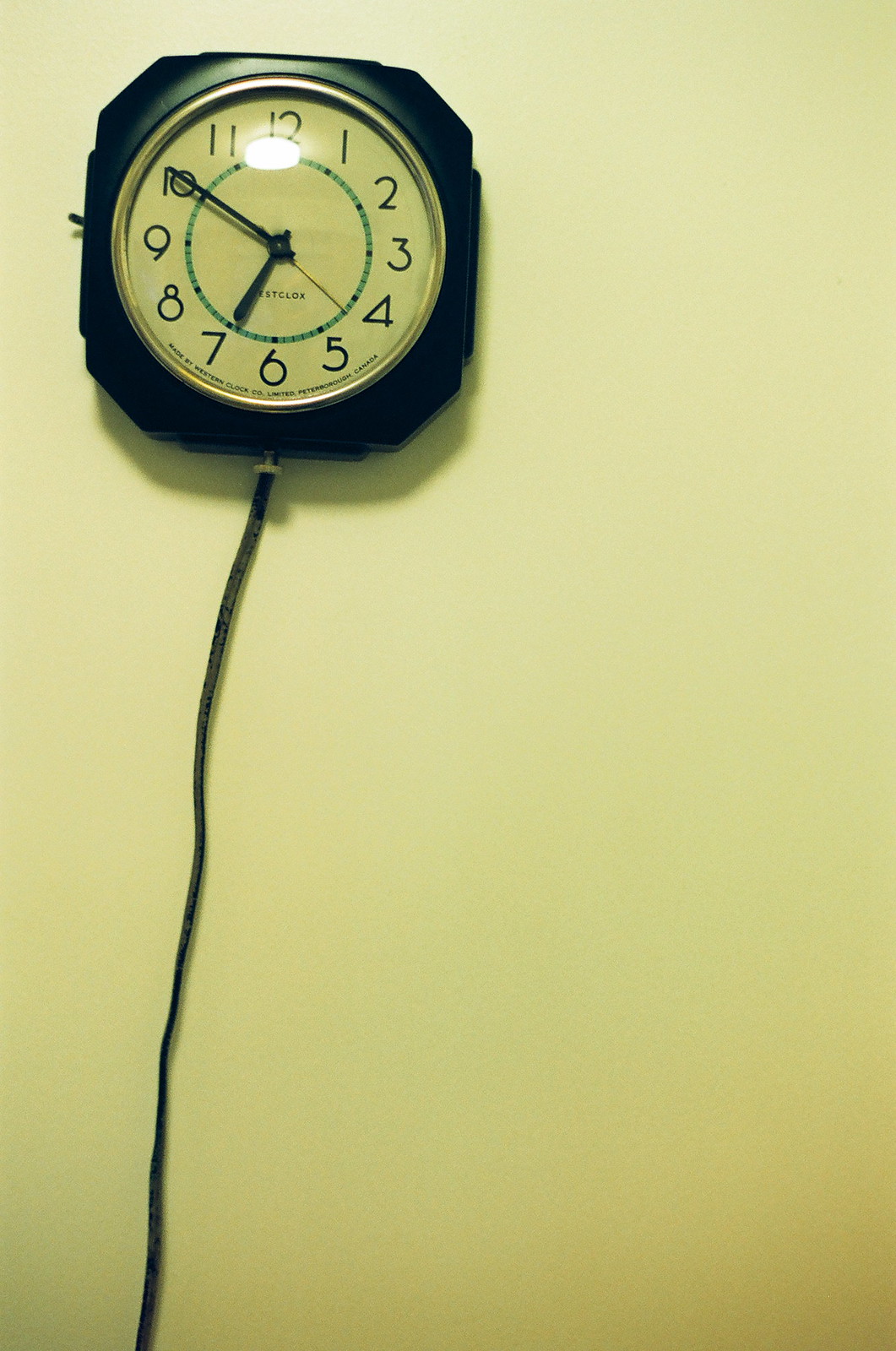A black wall clock, prominently positioned in the upper left-hand corner of the photograph, dominates the frame. The overall image possesses a yellow tint, resembling an Instagram filter, applied over what appears to be a white wall. This square-shaped clock has a sleek black plastic frame and features a silver rim encircling the round clock face. The clock face is protected by a clear plastic dome, through which the numbers 1 to 12 are visible. There is a smaller inner ring, marked with green and adorned with black dashes, indicating seconds and minutes.

The brand, "Westclox," is clearly printed just above the 6, nestled between this numeral and the center where the hands gather. The time on the clock reads 6:50, with the hour hand approaching the 7, the minute hand at the 10, and the second hand pointing precisely between the 4 and the 5. Extending from the base of the clock is a long black plastic electrical cord, which connects via a small silver attachment and trails out of the frame, suggesting it is plugged into a socket at the lower portion of the wall.